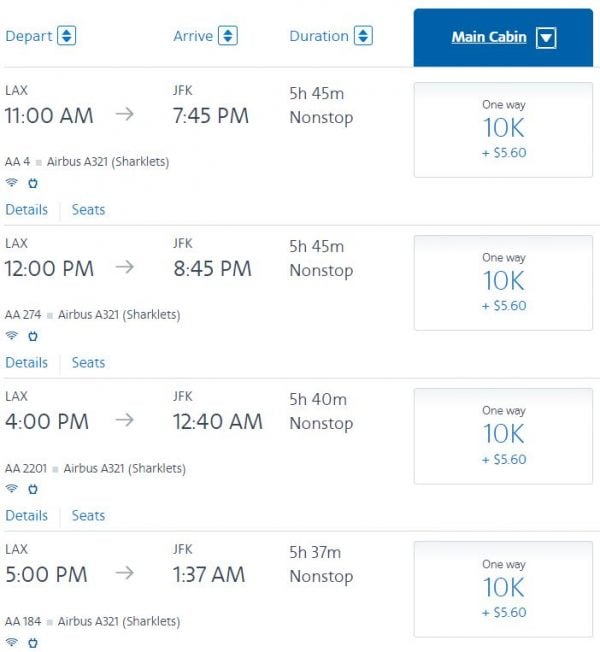Screenshot of a flight booking website showing various flight options in a detailed table. The table is categorized into four headings: "Depart," "Arrive," "Duration," and "Main Cabin," the latter being highlighted in a blue box with white font, indicating the seating option selected. The background is predominantly white, while the "Depart," "Arrive," and "Duration" headers are written in blue font, accompanied by arrows for adjusting search preferences.

The table displays four different flight results. Each result provides comprehensive information, including the departure and arrival times, specific departure and arrival locations, and the duration of the flight. Additional details are provided regarding the type of aircraft, availability of Wi-Fi, and charging outlets. Below each flight option, there are sections labeled "Details" and "Seats." On the far right of each row, the total cost for a one-way trip is displayed.